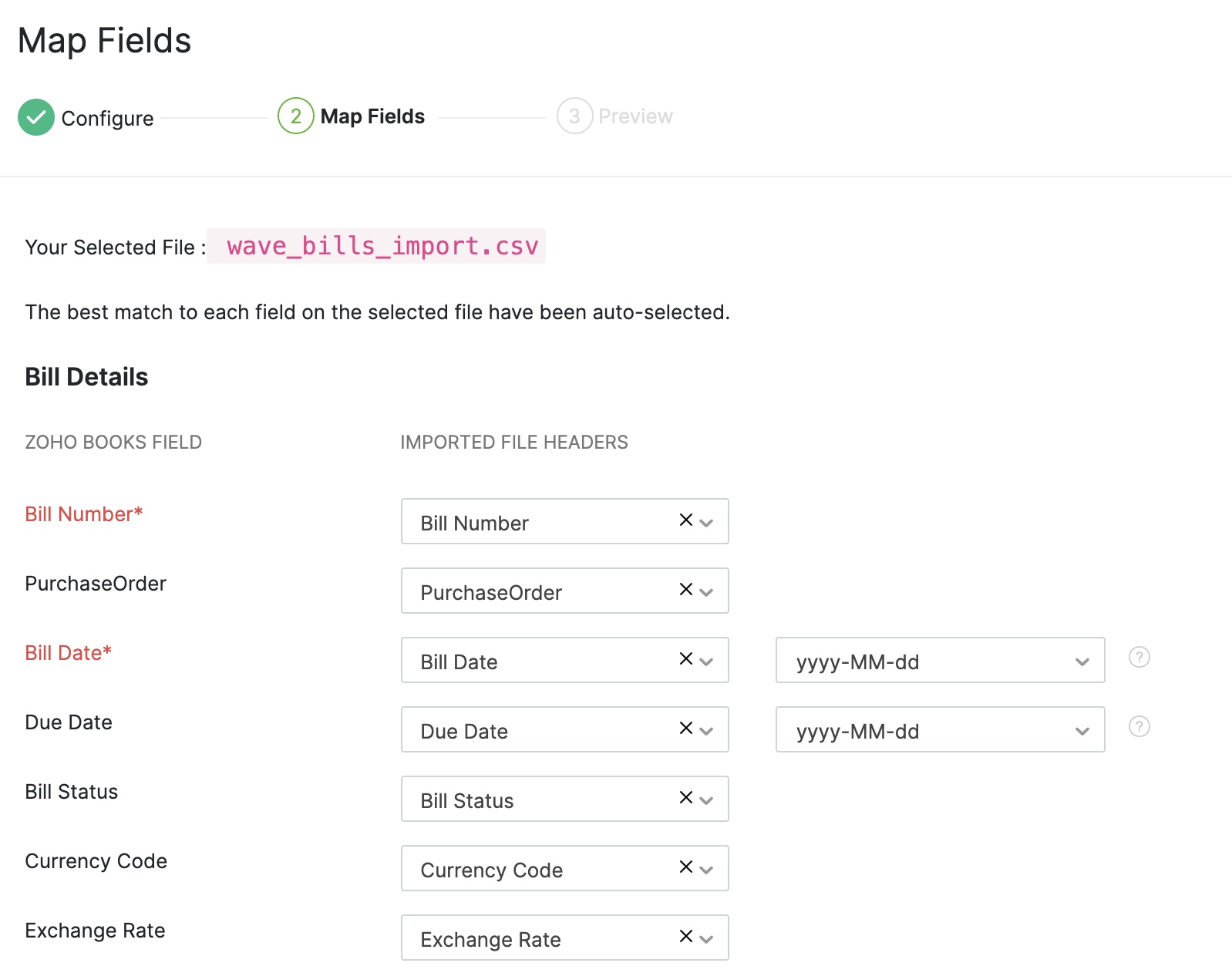The screenshot captures a form interface, structured in a step-by-step process for configuring and mapping fields for data import. At the top, the title "Map Fields" is prominently displayed in black font. Below this title, there is a green circle with a white checkmark inside, accompanied by the word "Configure." This is followed by a light gray horizontal line.

Progressing down, there is a white circle outlined in green with a green number "2" in the center. Next to this circle, in bold text, is the phrase "Map Fields." Continuing below is another horizontal line, followed by a light gray circle outlined in light gray, containing a light gray number "3." Adjacent to this circle, also in light gray font, is the text "Preview."

Another light gray line follows, below which the phrase "Your selected file:" appears in black font. Highlighted in bright pink font with a light pink background, the file name "wave_bills_import.cbs" is clearly displayed.

Further down, a guiding statement in black font reads, "The best match to each field on the selected file have been auto selected." Below this statement, the section labeled "Build Details" is written in bold black font. Underneath, the labels "Zoho Books Field" and "Imported File Headers" are displayed in light gray font. The latter label is also capitalized.

Subsequent fields are listed with their corresponding options. "Bill Number," noted in red font, has a corresponding drop-down box on the right labeled "Bill Number" with an X to indicate a selection. The same format is applied to "Purchase Order," written in black font with its selection box labeled "Purchase Order" including an X. The field "Bill Date," also in red font, is paired with a selection box on the right showcasing the label "Bill Date" with an X, accompanied by a separate drop-down box for the date format "YYYY-MM-DD."

Additional fields, such as "Due Date," "Bill Status," "Currency Code," and "Exchange Rate," are listed subsequently without specific details on their corresponding input mechanisms in this screenshot.